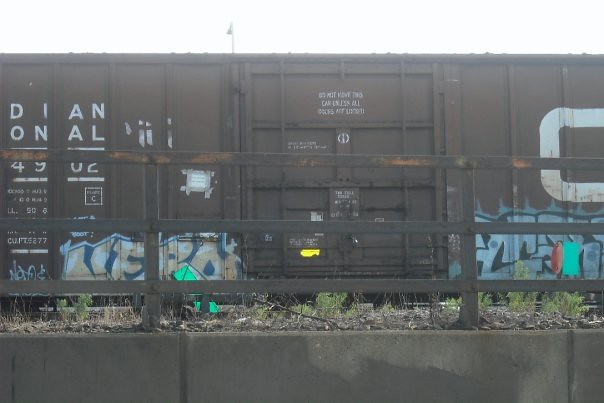The image depicts a brown train car, primarily metal, with visible areas of rust, positioned behind a concrete barrier and a black steel fence. The fence consists of vertical poles and three horizontal bars, showing signs of wear. In front of the fence is a small patch of dirt and grass, though the grass appears to be dying. The train car features prominent white text, including "DIANONAL" and the numbers "4902," positioned above a large central loading door. Smaller white text and horizontal lines can also be seen. The bottom of the train car displays graffiti in block-like letters, primarily in white with black borders, resembling the word "HERO." Above this graffiti, there's a taped area with some white markings inside. The overall scene is set against a clear sky.